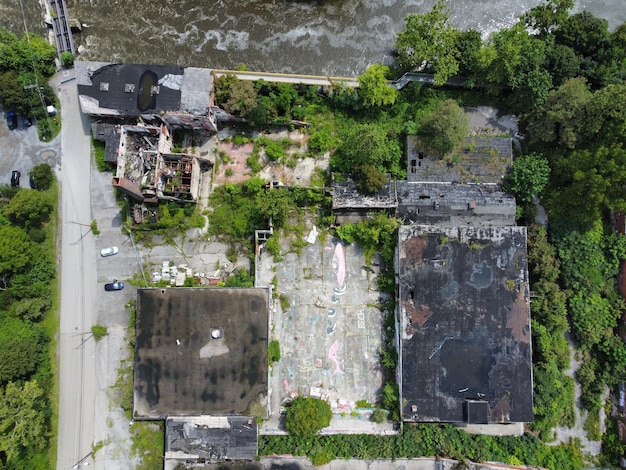This aerial photograph, possibly taken from Google Maps or a satellite view, captures a deteriorating property surrounded by lush greenery. Central to the image is a large building on the right, notable for its patchy roof in varying shades of brown, black, and gray, suggesting significant wear and deterioration. Adjacent to this, smaller parking lots hold a couple of cars—a white one and a blue one. To the left, there is a house-like structure that appears roofless and open, presenting a stark contrast to the surrounding structures. Below, another large building mirrors the state of the first, with its roof similarly in disrepair. At the top of the image, there's a suggestion of water, possibly a river or lake, adding an element of ambiguity due to the nature of satellite imagery. The entire area is framed by dense trees, enhancing the sense of isolation and neglect. Additionally, a road runs to the left of the property with more trees past it, and a bridge is visible in the upper left corner.